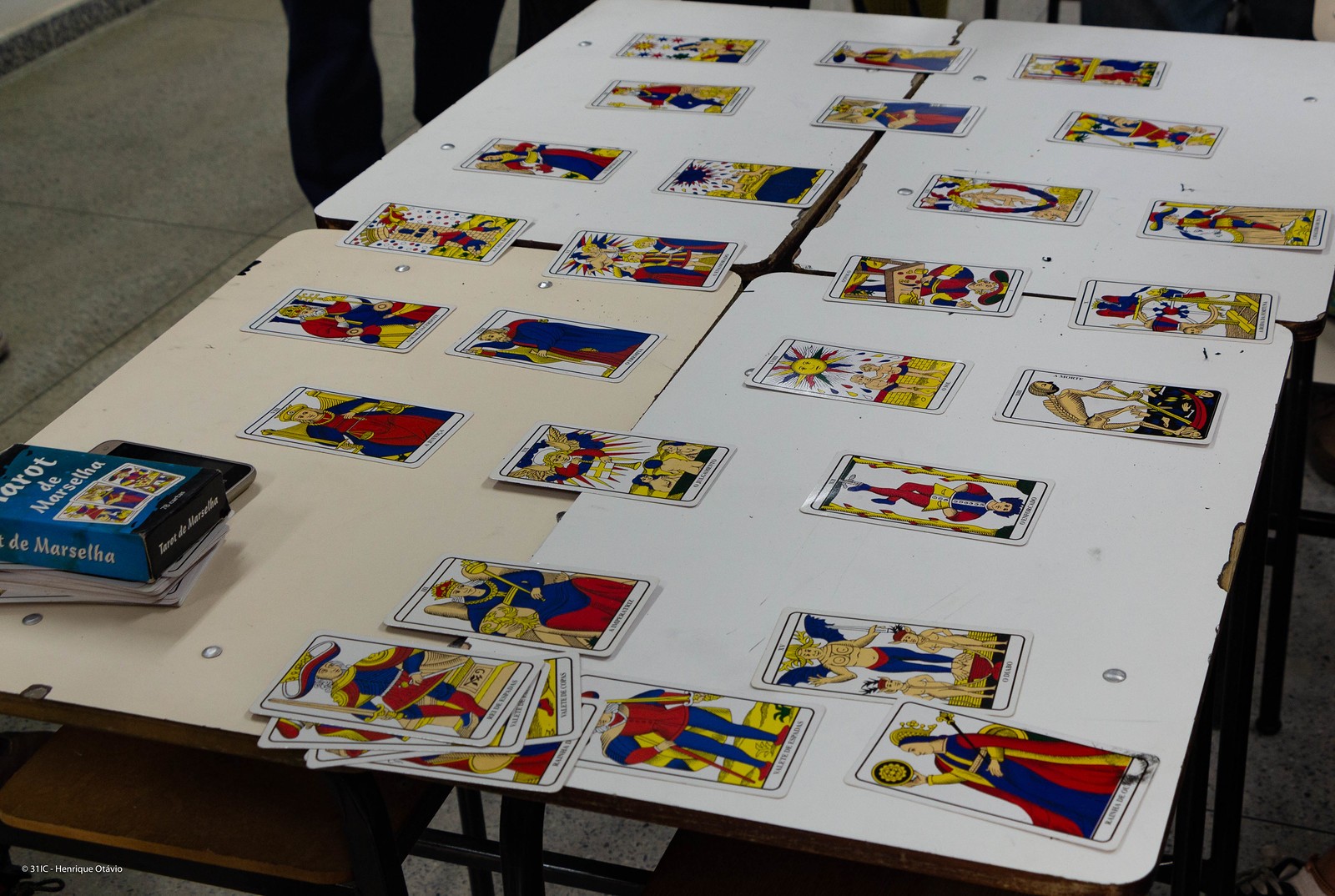In the photograph, you are seen examining an assortment of tarot reading cards. The layout spans across four white rectangular tables that have been pushed together to form one large surface. Notably, one of the tables stands out with a yellowish tint, contrasting against the predominantly white tables. These tables show clear signs of wear and tear, with chipped paint and missing sections, suggesting they are quite old and well-used.

The tarot cards are spread out across the tables in a seemingly random fashion, covering nearly the entire surface area. In the bottom left-hand corner of the image, a box labeled "Tarot" confirms the nature of the cards. In front of the tables, closest to the person taking the photograph, there is a pile of additional tarot cards that appear to have been set aside, possibly not needed for whatever reading or display is taking place.

Additionally, in the upper left corner of the image, some legs are visible, indicating the presence of other people—perhaps an audience or participants in a fair, eager to see the tarot card readings. The overall scene conveys a sense of curiosity and exploration of the mystical world of tarot, set against the backdrop of these well-worn tables.